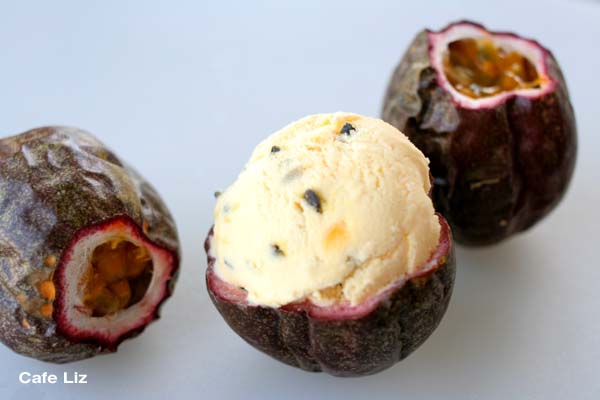In the photograph, three round, brownish-maroon objects that appear to be figs or a similar type of fruit are prominently displayed. The image is horizontally oriented with three of these fruits arranged from left to right. The fruit on the left, partially out of the frame and lying on its side, reveals an interior filled with a gooey orange substance and tiny seeds, encircled by a white layer and bordered with red. 

The fruit on the upper right stands upright, its blurry top showing a similar orange, seed-filled center surrounded by white and red, set against the brown outer skin. In the center and in sharp focus, a halved fruit showcases its cross-section, highlighting the pink and white perimeter and a scoop of white ice cream in its core. The ice cream appears to be vanilla with specks of chocolate and possibly tiny seeds or fruit pieces, adding texture and visual interest. There's a hint of orange at the bottom of the ice cream, indicating it might be infused with segments or flavors related to the fruit. 

The photograph's bottom left corner features the text "Cafe Liz" in white, suggesting it might be a menu item or featured dessert from this establishment.